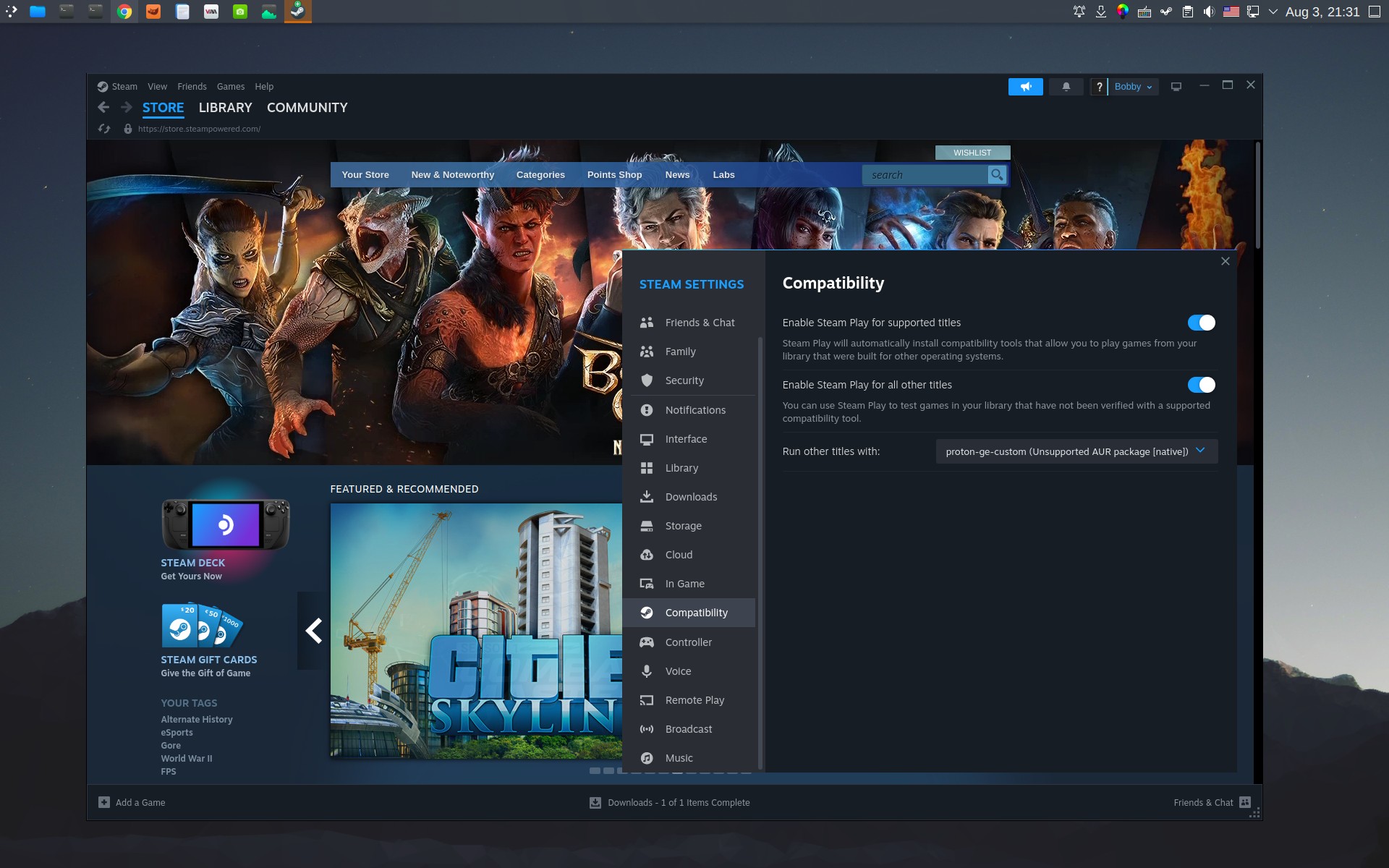A screenshot of a website promoting video games is displayed on a computer screen. The website features a large, vivid image prominently showcasing various in-game characters in vibrant colors such as reds, blues, greens, and grays. In the upper left-hand corner of the screen, navigation tabs labeled "Store," "Library," and "Community" are visible. 

Overlaying the characters, a pop-up window titled "Stream Settings" appears, with a vertical section detailing numerous streaming configuration options. There's also a partially readable section that references a compatibility page with the word "Explore," though the text is too small to be clearly deciphered. 

In the background, the clear desktop shows a screensaver of sky and mountains, along with standard computer icons along the top edge of the screen. Additionally, in the bottom left corner of the screenshot, a section illustrates a vibrant image of a skyscraper labeled "City Skyline." Adjacent to this is a brightly colored television icon with the label "Stream Check" in purple and white. Below this, there are three blue boxes.